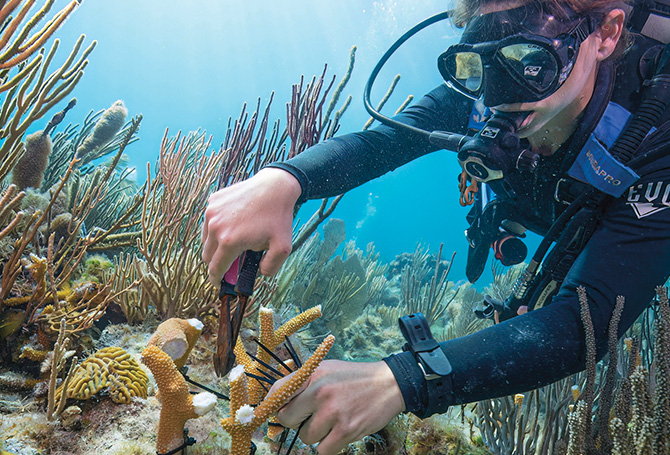The image depicts a person underwater in very clear, light blue water, dressed in complete scuba gear, including a black wetsuit, diving mask with a mouthpiece, and diving cylinders. They are holding a pair of clippers and appear to be engaged in clipping or trimming corals. The scuba diver is focused on a beige branch-like coral structure in front of them, using their tools to carefully trim the coral. Surrounding them are various colorful corals, including orange, yellow, and green, and different aquatic plants, suggesting a vibrant tropical setting. The diver also has a watch on their left wrist, which is visible along with their face and arms as they work intently on maintaining the underwater coral environment.